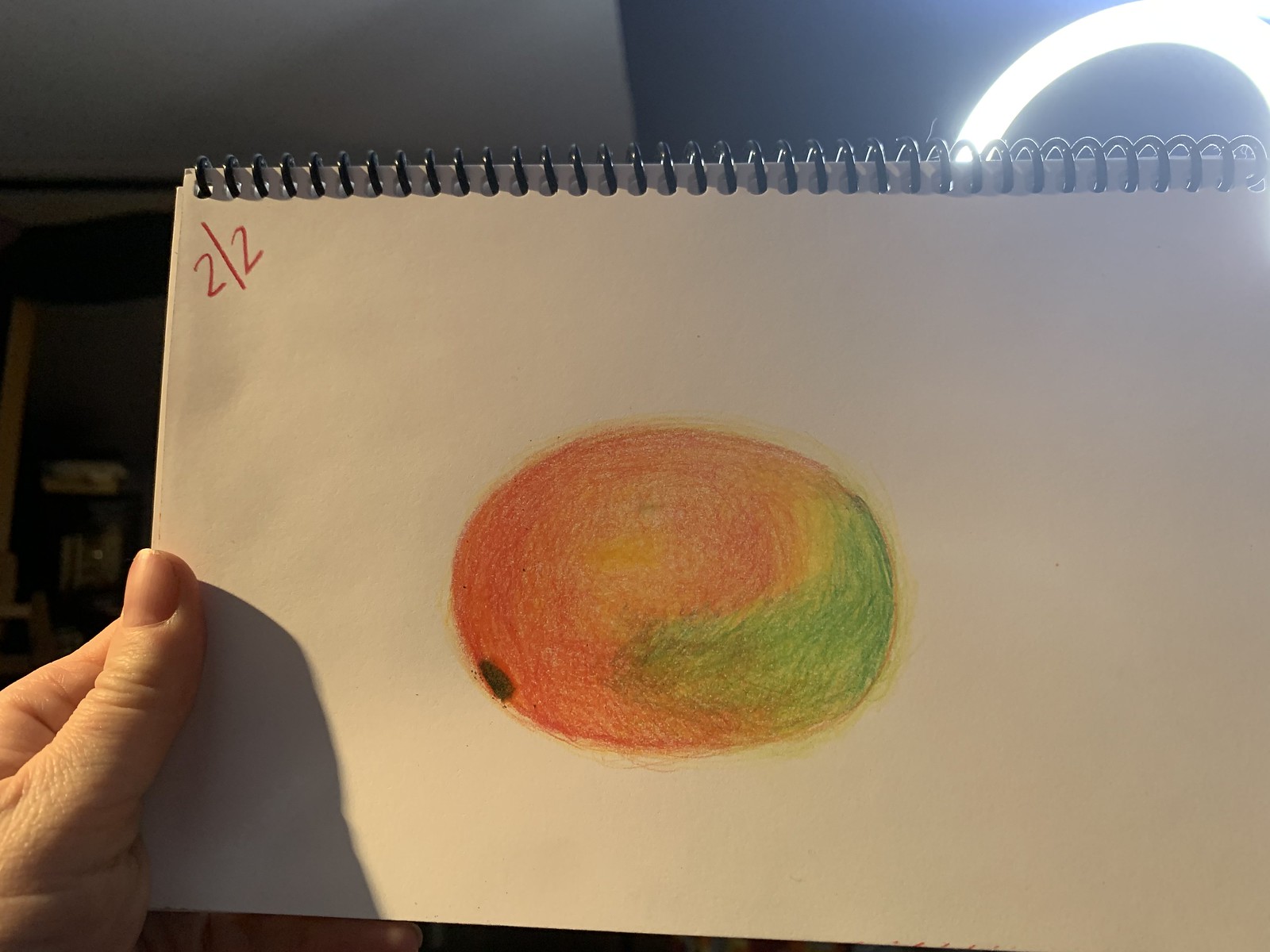A detailed sketch rendered in pastel pencils depicts an oblong peach that appears slightly misshapen. The peach showcases a gradient of peachy orange hues on the left and subtle hints of green on the right. The artwork is created on a small, spiral-bound sketch pad, with the spiral binding positioned at the top. The sketch pad is held by a person's left hand, partially obscuring the bottom. A mysterious notation, "2/2," is visible at the edge of the sketch, potentially indicating a date or another form of marking. The background features a contrast between a white and black wall, with a distinctive, whitish-blue neon loop adding an intriguing modern touch to the scene.